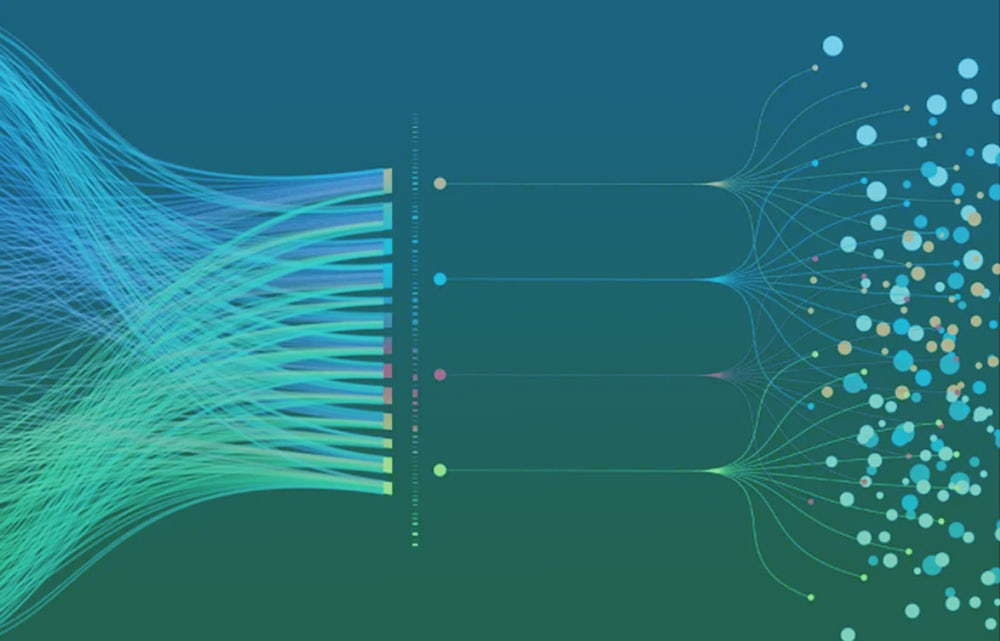This image appears to be an intricate, AI-generated drawing set against a dark blue background that transitions into varying shades of blue and green. The central motif consists of multiple abstract, spiraling lines resembling radiographs or sound waves. These lines converge towards the center, where they interact with four distinct dots—colored in white, blue, pink, and light green. Emerging from the center, these lines extend rightwards, culminating in small, colorful flares of blue, pale blue, brown, pink, and light green dots. The entire composition has an abstract, almost scientific feel, with no accompanying text to provide further context. The detailed depiction of strings and bubbles, alongside the interplay of vibrant colors on a predominantly blue backdrop, gives the piece a complex, yet harmonious appearance.